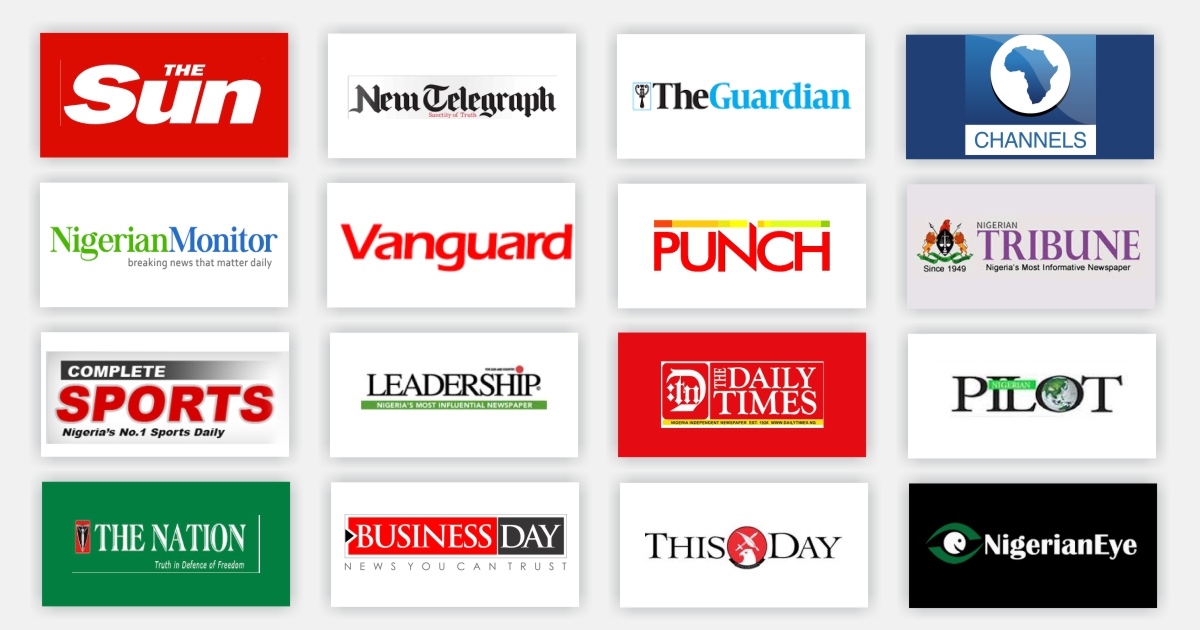The image displays 16 rectangular logos of various news outlets, predominantly from Nigeria. Each logo is unique, showcasing distinctive colors and designs:

1. **The Sun**: Featuring a striking red background.
2. **New Telegraph**: Displayed in black with an old-fashioned font on a white background.
3. **The Guardian**: Highlighted with a light blue logo on a white background with "The" in black.
4. **Channels**: Incorporating an image that resembles the African continent.
5. **Nigerian Monitor**: Displayed in light blue with white beneath it.
6. **Complete Sports**: Another news logo, but specific details are omitted.
7. **The Nation**: Positioned beneath the "New Telegraph" logo.
8. **Vanguard**: Located next to "Complete Sports."
9. **Leadership**: Appearing beneath the "Vanguard" logo.
10. **Business Day**: Found below the "Leadership" logo.
11. **Punch**: Positioned beneath the "Guardian" logo.
12. **Daily Times**: Immediately below "Punch."
13. **ThisDay**: Located beneath "Daily Times."
14. **Tribune**: Situated below the "Channels" logo.
15. **Nigerian Tribune**: Listed directly beneath "Tribune."
16. **Pilot**: Found next to "Nigerian Tribune."

All outlets are news-related, emphasizing their significant presence within Nigerian media landscape.